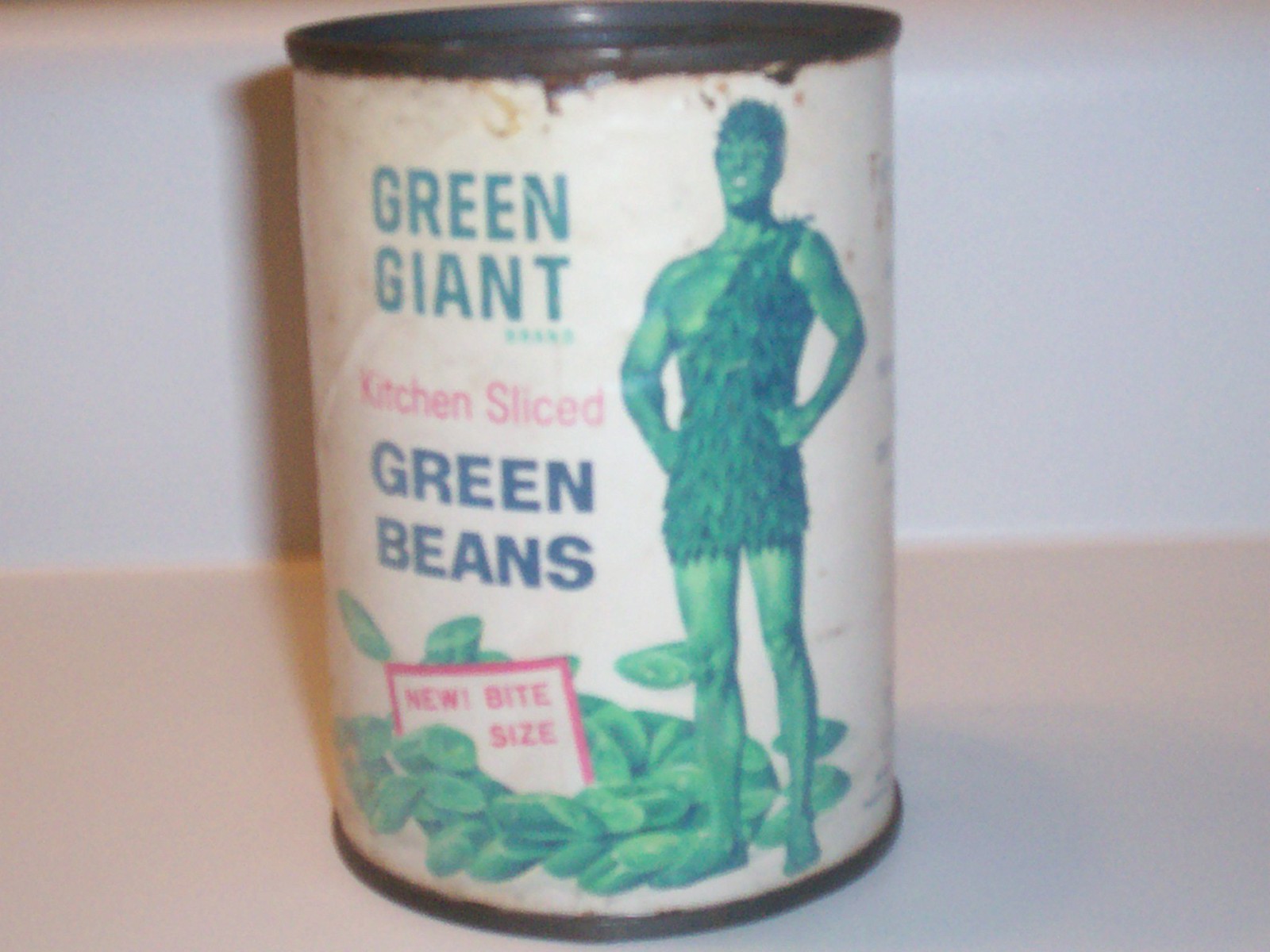This photograph depicts a vintage-looking can of Green Giant green beans, set against a white wall and resting on a flat, beige surface. The cylindrical can features a white product label marred by age. The label prominently displays the Green Giant brand name in green text at the top, followed by "Kitchen Sliced" in pink text, and "Green Beans" in blue text. To the right of these text elements, the iconic Green Giant mascot is visible as a green-skinned figure wearing a leafy outfit. Below the text is an illustration of a pile of green beans, along with a white and pink sign that reads "New Bite Size" in pink text. The can's structure includes a dark brown ring at both the top and bottom, further emphasizing its aged appearance. The overall ambiance of the photo, with its plain white wall and flat surface, highlights the nostalgic and worn nature of the can.